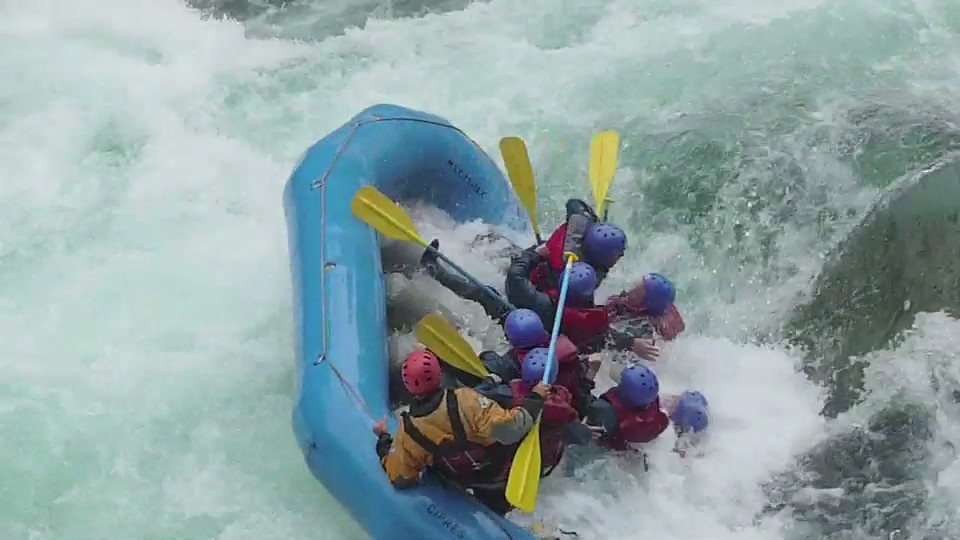The image captures a thrilling moment of a whitewater rafting adventure with eight visible participants, although there may be a hidden ninth person. All are geared up for outdoor activity, wearing windbreaker-type jackets and helmets—one red and the rest blue or purple. They are in an inflatable blue raft navigating through fierce, choppy waters full of white foam from the crashing waves. The raft is tilting precariously to the right, and some rafters have already fallen into the turbulent, greenish water, while others are desperately clambering up the higher side to stay aboard. The instructor, distinguishable by a red helmet and possibly an orange or brown jacket, is positioned at the end of the raft. They all clutch yellow paddles with turquoise poles, battling to regain control amidst the chaos.